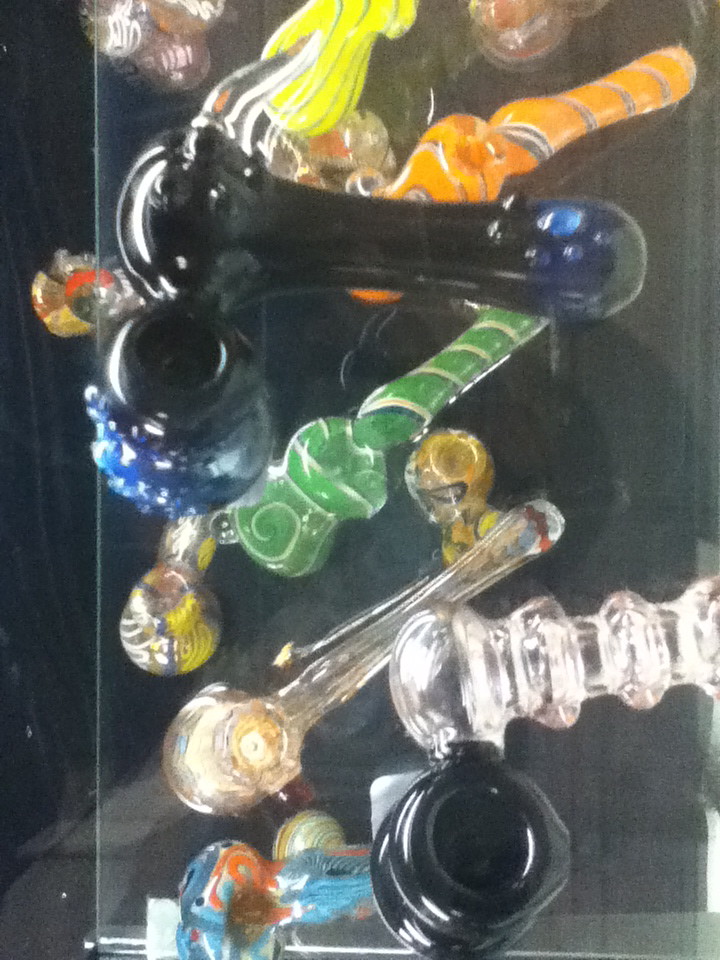This image showcases a block transparent case containing a variety of colorful, intricately designed glass objects resembling jellyfish or tadpole-like figurines. These objects, suspended as if floating, create the illusion of movement within the translucent casing, despite being static. Positioned at various levels, the case features a blue figurine at the bottom, followed by a clear one, then a green, an orange, and finally a yellow one towards the top, giving an impression of an underwater scene. The foreground displays a cylindrical-shaped glass pipe with a bulbous end and an upward-facing bowl, accompanied by a small hole at the opposite end. Surrounding this central piece, other similarly designed glass pipes in various colors—yellow, orange, green—add to the collection’s vibrancy. Notably, a larger ribbed pipe in black and clear hues prominently stands out in the bottom right corner.